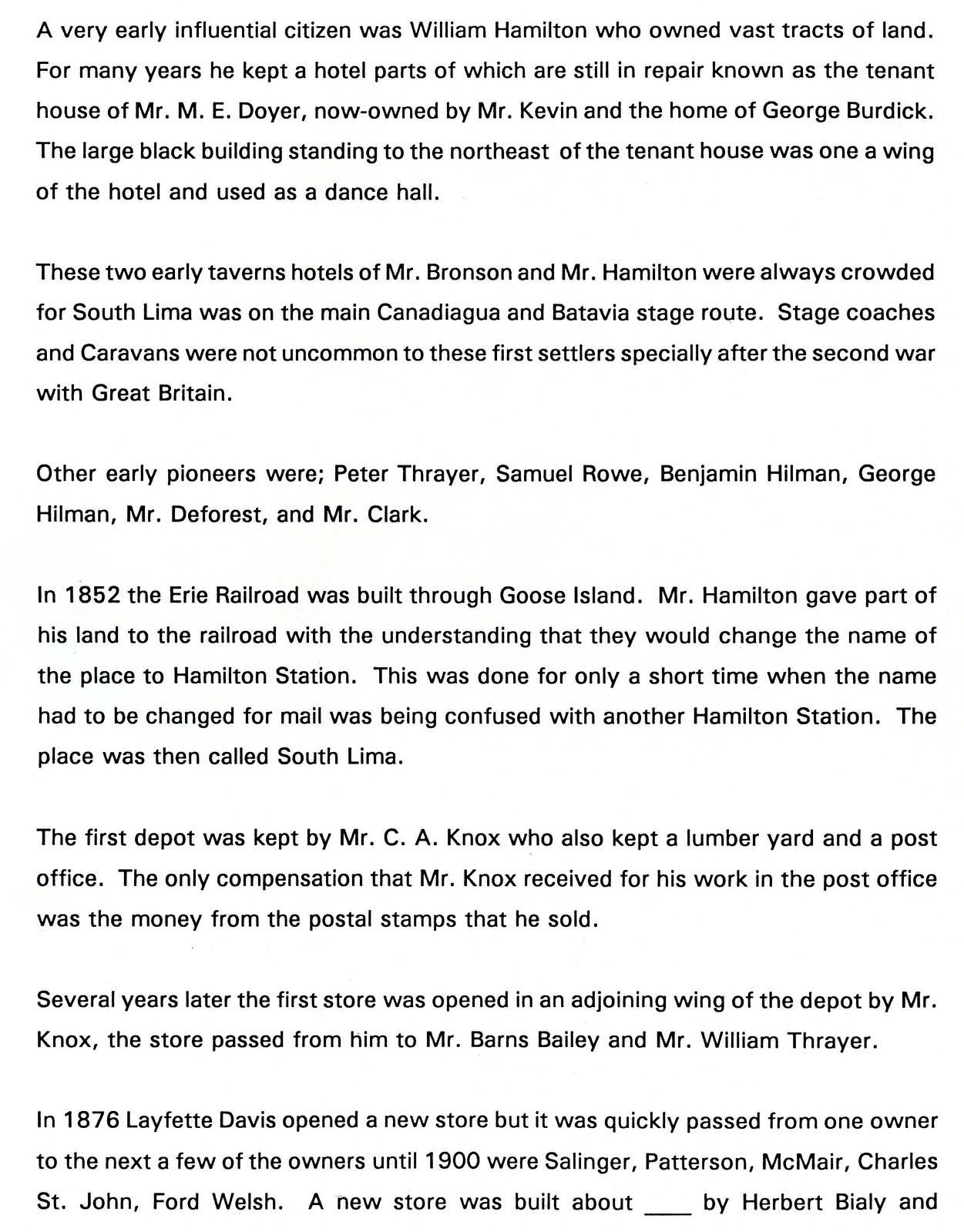This vertically oriented image features seven paragraphs of black text on a white background, most likely historical data. The text begins by highlighting an early influential citizen named William Hamilton, who owned vast tracts of land. He maintained a hotel for many years, parts of which still exist and are known as the tenant house of Mr. M. E. Dower, now owned by Mr. Kevin and serving as the home of George Burdick. Another notable structure is a large black building to the northeast of the tenant house, which was once a wing of the hotel used as a dance hall. These two early taverns, operated by Mr. Bronson and Mr. Hamilton, were popular due to South Lima's location on the main Canandaigua and Batavia stage route, a key passageway frequented by stagecoaches and caravans, especially after the Second War with Great Britain.

Subsequent paragraphs detail other early pioneers such as Peter Thayer, Samuel Rowe, Benjamin Hillman, George Hillman, Mr. De Forest, and Mr. Clark. In 1852, the Erie Railroad was constructed through Goose Island, and Hamilton donated part of his land for the project under the condition that the area be renamed Hamilton Station. However, due to confusion with another Hamilton Station, it was later renamed South Lima. The first depot was managed by Mr. C. A. Knox, who also ran a lumber yard and a post office, earning his compensation through the sale of postal stamps. Knox later opened the first store in an adjoining depot wing, which eventually passed to Mr. Barnes Bailey and Mr. William Thrayer. In 1876, a new store was opened by Lafayette Davis, but it changed hands frequently among owners such as Salinger, Patterson, McMayor, Charles St. John, and Ford Welsh. A new store was eventually built by Herbert Bialy.